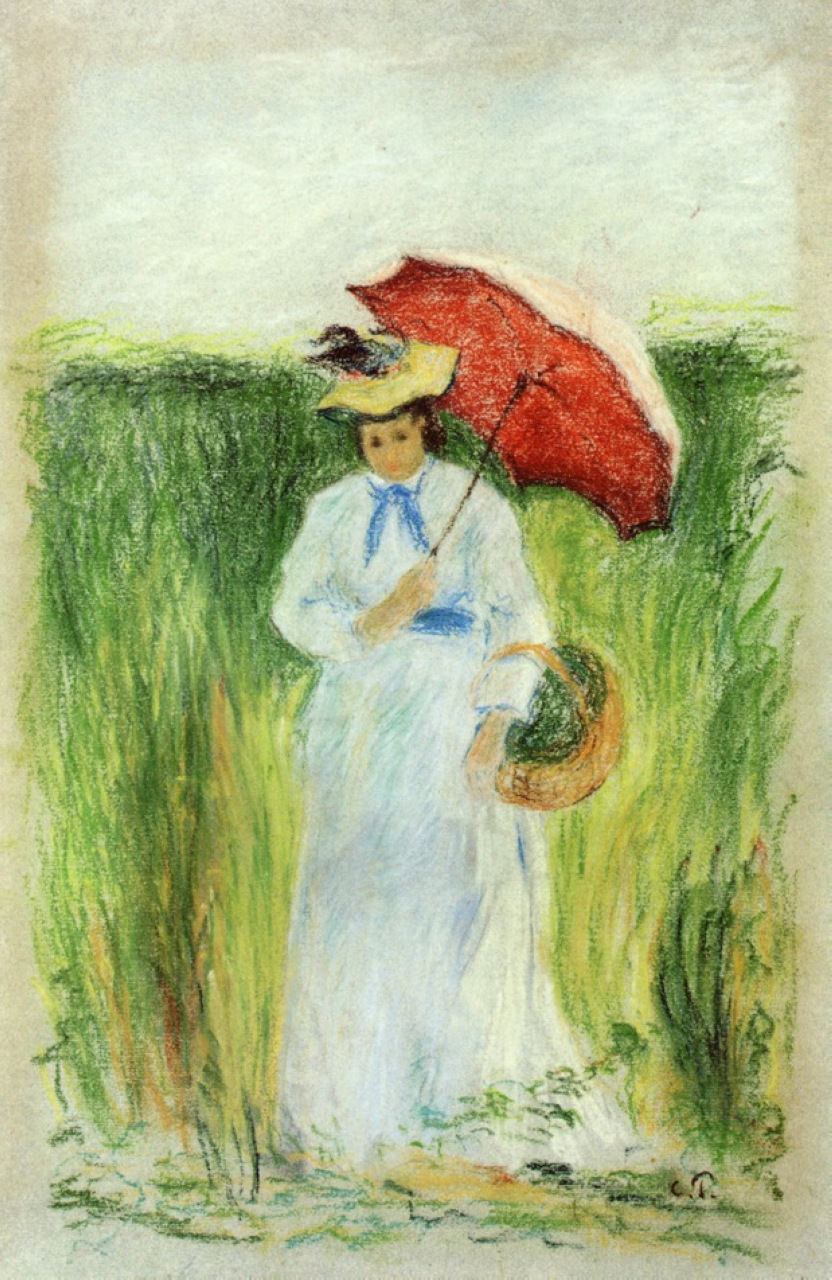This is a detailed colored pencil drawing with a hint of crayon or pastel, showcasing a woman walking outdoors. She is dressed in a long, flowing white dress with a blue belt and a blue scarf around her neck. Adorning her head is a light-colored bonnet, accented with some feathers, adding a delicate touch. With her left arm, she gracefully carries a basket filled with green vegetation, suggesting she has been gathering flowers or plants. In her right hand, she holds an eye-catching parasol, striking with its red and white contrast, likely used for protection from the sun as the bright day doesn't suggest rain. She is surrounded by tall green grass, which stretches into the background, and the sky above is depicted in a soft, white hue. The overall style of the drawing is impressionistic and somewhat loose, with aged paper adding a timeless quality to the artwork. The drawing’s colorful and sensitive approach vividly captures a serene moment outdoors.